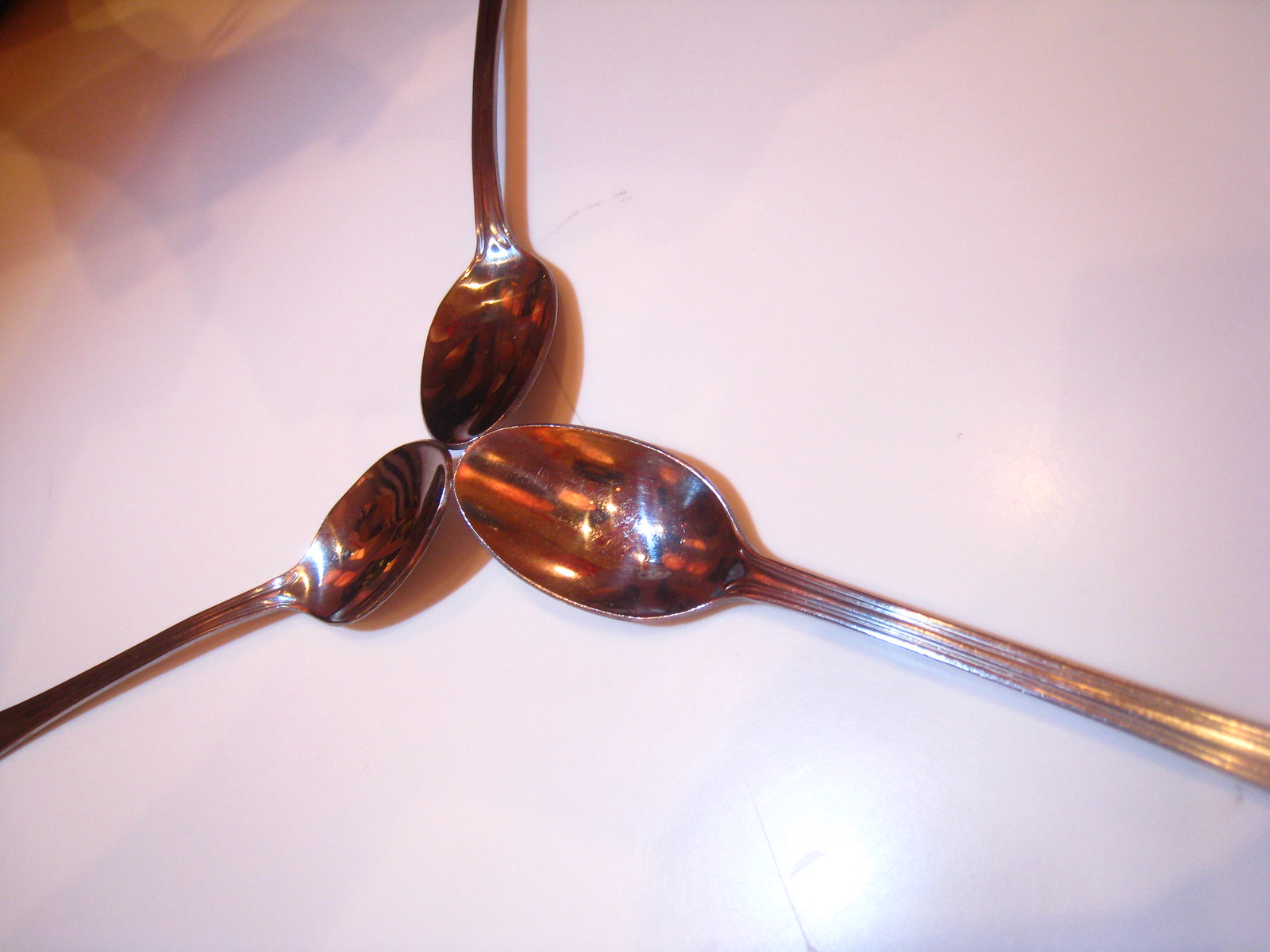The photo features three shiny silver spoons arranged in a triangular formation, with their tips touching and their handles extending outwards at 120-degree angles from each other. The spoons are positioned on a white table, which has a pinkish tinge likely due to poor color correction in the image. Though the spoons appear to have a rose gold hue, this is probably an artifact of the tint problem. The design of the spoons is plain and simple, and they feature notably long handles.